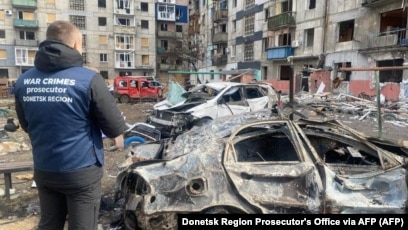In this color landscape photograph, a war-torn scene unfolds in a dilapidated dirt parking lot, evidently part of a conflicted downtown area. The central subjects are several severely damaged vehicles, with the two most prominent cars—a gray one with bashed-in side doors and a missing fuel door, and a white one behind it—both appearing totaled. The vehicles are rusted and dilapidated, reinforcing the chaotic ambiance. A man stands on the left in a black hoodie layered with a blue vest, his back to the viewer. Emblazoned on his vest are the words "War Crimes Prosecutor," suggesting his grim task of inspecting the wartime wreckage before him. Behind the cars, a decrepit, multi-story apartment or commercial building, with walls appearing bombed-out and weathered, adds to the sense of devastation. The image bears a black horizontal stripe at the bottom right corner with white text that reads "Donetsk Region Prosecutor's Office via AFP (AFP)."